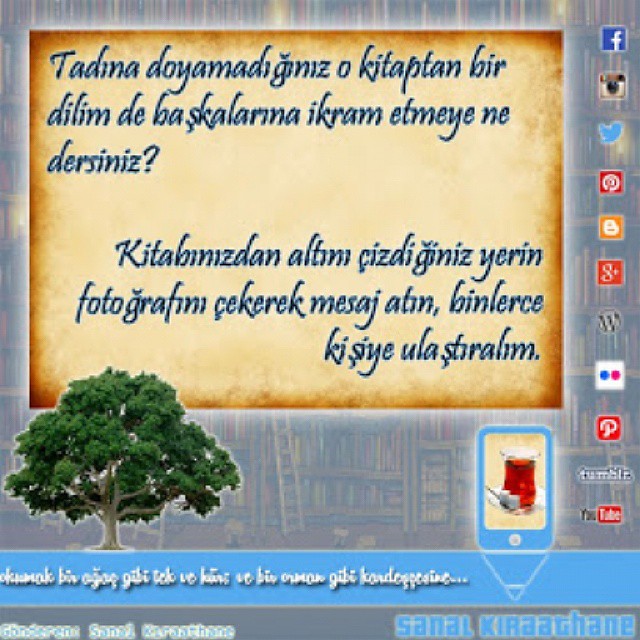The image depicts a square-shaped flyer that combines elements of a recipe and an advertisement, primarily written in an Indian language. The text, composed in dark blue font on a light brown background, features several statements in this foreign language, with two prominent sentences—one at the top and another at the bottom. On the left side of the flyer, beneath the text, there is a vibrant, large green tree, adding a touch of nature to the design. The bottom of the flyer also showcases a picture of a glass of tea accompanied by a couple of sugar cubes. The right-hand border of the flyer features a vertical line of small social media icons, including Facebook, Instagram, Twitter, Pinterest, Google+, Tumblr, and YouTube, indicating various ways to connect with the company. Faintly visible in the background of the flyer is an image resembling a library, adding an additional layer of depth to the visual. The overall color scheme is dominated by blue and light brown tones.